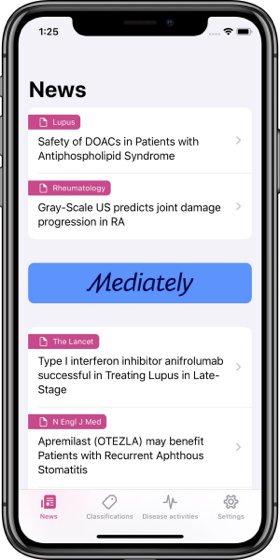The image is a vertically oriented picture of a black-rimmed smartphone. The screen displays a gray background with various sections of text and icons. At the top left corner, the time is shown in bold black text as "1:25," while the top right corner features the signal strength bars, a Wi-Fi icon, and a battery life icon.

Beneath this header, the word "News" appears prominently in bold black text. The screen displays several white horizontal rectangular boxes containing headings and brief descriptions. 

One box features the word "LUPUS" in a mauve color, followed by the text "Safety of DOACs in patients with antiphospholipid syndrome" in black. Another box titled "RHEUMATOLOGY" in mauve color includes the text "Grayscale US predicts joint damage progression in RA" in black. 

A distinctive blue horizontal box contains the word "IMMEDIATELY" in black text.

Further down, additional white boxes with mauve headings include "The Lancet: Type 1 interferon inhibitor anifrolumab successful in treating lupus in late stage" and "N Engl J Med: Apremilast may benefit patients with recurrent aphthous stomatitis."

At the bottom of the screen, there are navigational options labeled "News," "Classifications," "Disease Activities," and "Settings," with "News" highlighted to indicate the current selection.